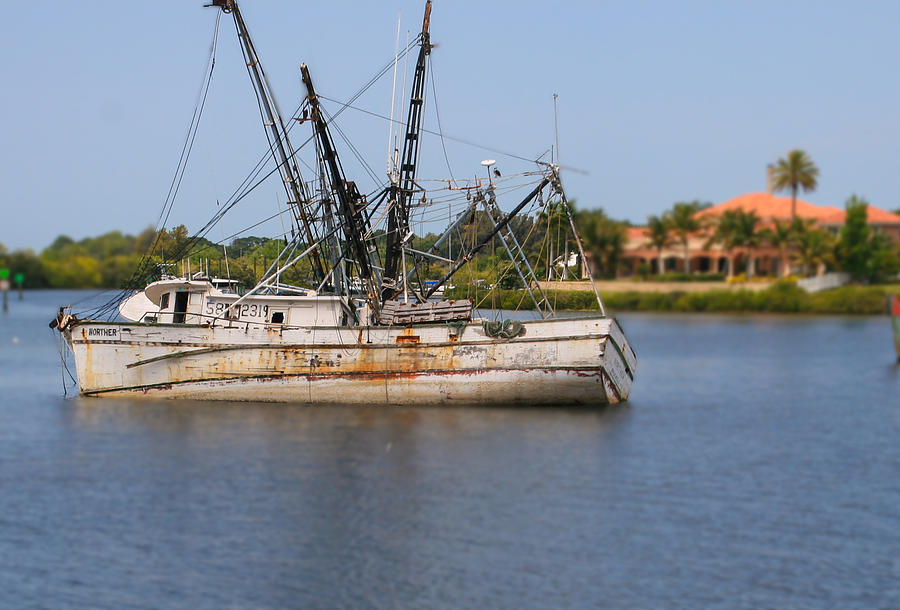In a serene tropical or subtropical setting, a rusty, gray and white fishing vessel dominates the scene, listing noticeably to the right as if it may be sinking or in need of assistance. The boat is covered with rigging for nets, lines, ladders, and various equipment, adding a busy complexity to its worn appearance. On its hull are faint, hard-to-read numbers and markings. The vessel is set against bright blue, calm waters that reflect the sky and a lush, vibrant green landscape. In the background, a house with white walls and an orange, possibly terracotta roof, reminiscent of South Florida architecture, stands near the shore. The house has multiple windows and prominent front columns, further adorned by a standout palm tree amidst thick, luxuriant vegetation.